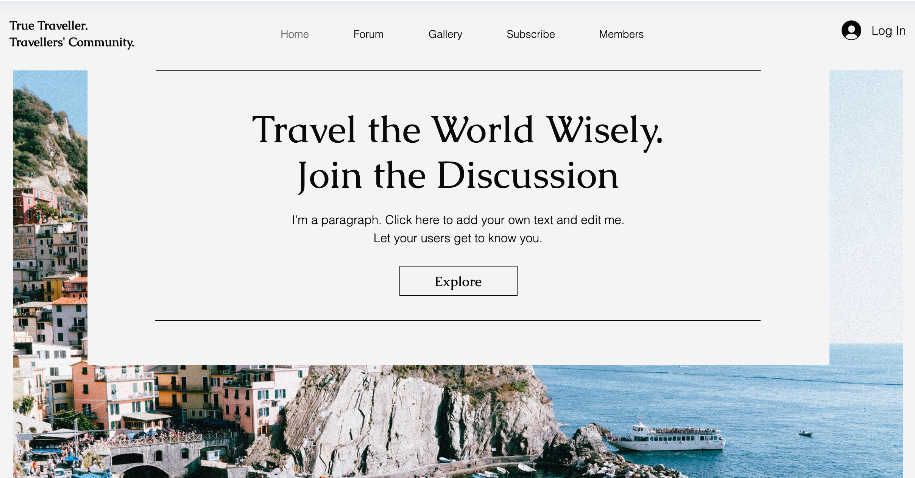The image showcases a serene and stunning landscape against a light blue backdrop. At the top, the title "True Traveler and Travelers Community" is prominently displayed. Below this title, there is a navigation bar featuring options such as Home, Forum, Gallery, Subscribe, and Members, alongside a circular icon indicating the login area. The page includes a larger light blue box with bold text that reads "Travel the World Wisely. Join the Discussion." A placeholder paragraph follows, encouraging users to add their own text and inviting others to learn more about the community. An "Explore" button is positioned beneath this section.

Encircling these elements is a captivating photo of an idyllic, ancient city nestled on a mountainside. The city overlooks a vast and vividly blue ocean, with a majestic cruise ship and a smaller boat floating gracefully on the water's surface. The sky above is a clear, light blue, perfectly complementing the overall serene atmosphere. The city itself is adorned with stately, towering buildings climbing up a winding hill, interspersed with lush greenery. The entire scene exudes tranquility and beauty, making it an inviting visual for any traveler.